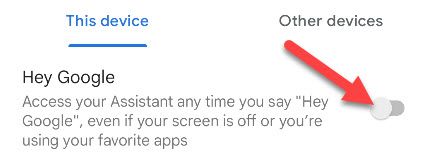The image features a minimalist design with a white background and blue, underlined text on the left-hand side that reads "This device." Adjacent to this, on the right-hand side, is gray text that says "Other devices." Below this section, on the left side, black text states "Hey, Google," followed by a gray description: "Access your assistant at any time. When you say, 'Hey, Google,' even if your screen is off or you're using your favorite apps." Beneath this text, there is a slider switch, currently positioned to the left and grayed out, indicating that it's off. A prominent red arrow from the upper left corner points directly at the switch. This is the entire content of the image, with no additional elements present.